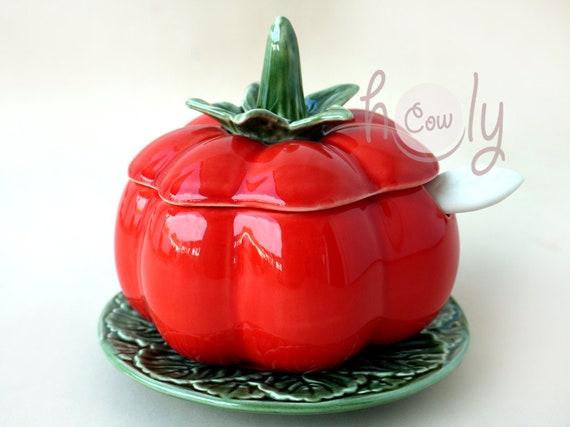The image depicts a shiny ceramic jar designed to resemble a tomato. The jar is vividly colored with a glossy red body featuring pronounced ridges. It has a matching lid adorned with a green stem and leaves jutting around it. The jar sits on an embossed green saucer with leaf-like petal details around its edges. In the top right corner of the image, "H-C-O-W-L-Y" is written in a circular arrangement on a bright white background. A small, white knob protrudes from the body of the tomato. The clear, close-up photo, taken in natural lighting, suggests this jar could be used for storing items like candies or keys.